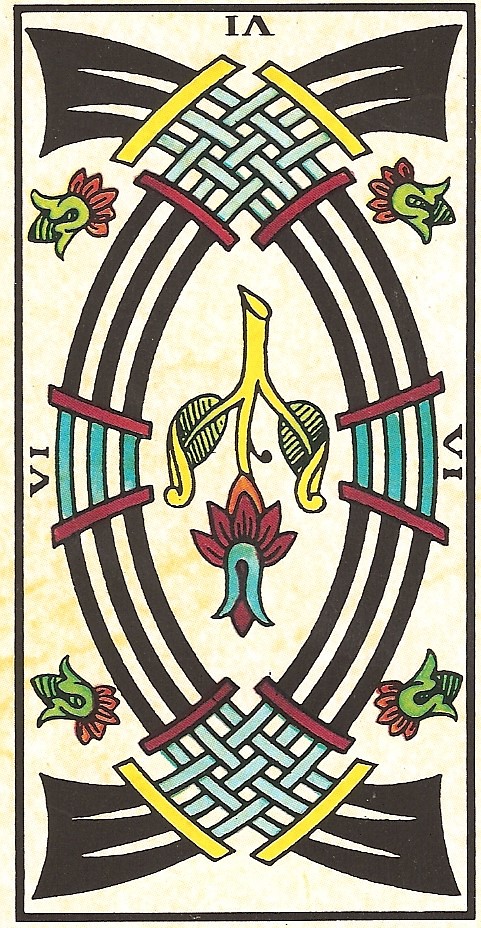The image is a long, rectangular, vertical composition that evokes the aesthetic of a tarot card. The background features a white and yellow pattern that resembles marble or a sponge-paint effect, adding a textured look. Along the sides of the image are four green flowers, shaped like tulips or bellflowers. These flowers showcase red petals emerging from their round, bell-like bases.

Two prominent black tribal-like stripes curve gracefully throughout the background, each stripe interspersed with two white lines, creating a visually striking contrast. The Roman numeral "VI" appears on either side of the image, while an inverted "VI" is positioned prominently at the top, adding a symmetrical element.

In the middle of the composition, blue cross-hatching overlays yellow rectangles, providing a stark contrast in color and texture. Additionally, there are red rectangles interspersed with areas of blue or teal, which contribute to the vibrant and dynamic color palette of the artwork. This intricate visual arrangement makes the piece both captivating and complex.